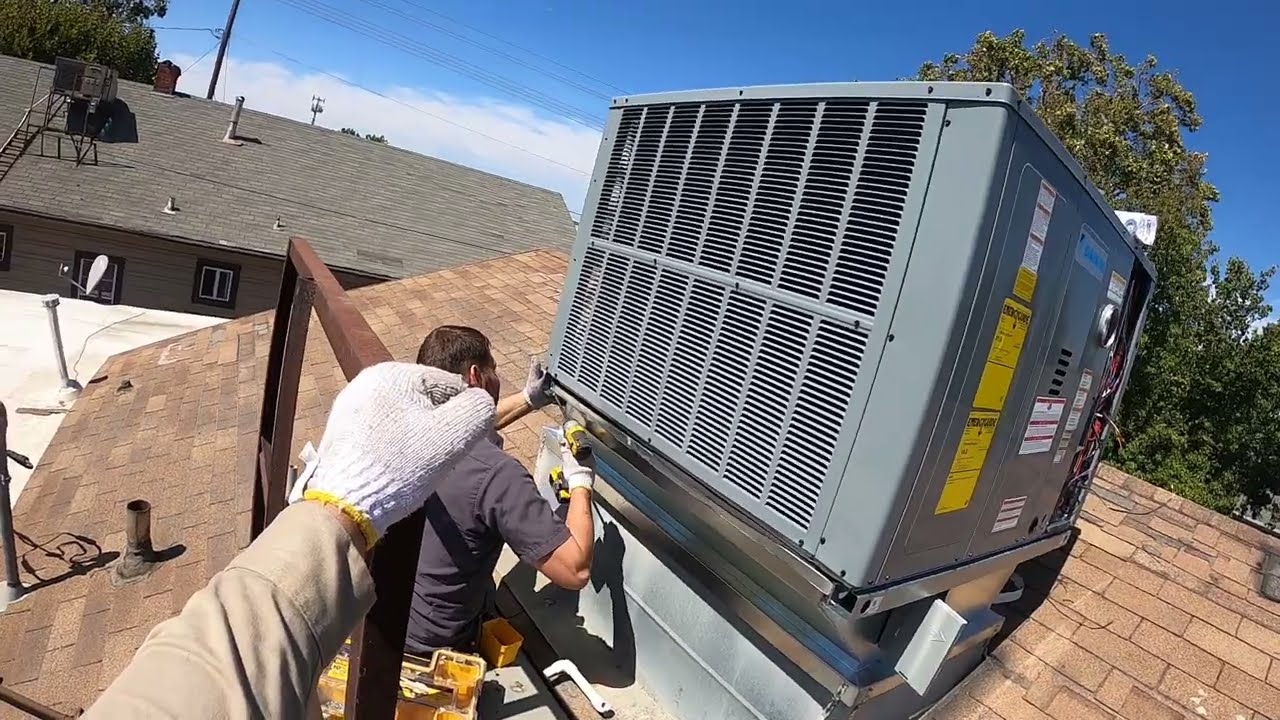This horizontally-aligned rectangular photograph captures a scene atop a slanting, light-to-medium brown shingled roof under a clear blue sky dotted with thin white clouds. In the upper left background, there's a house with a light gray roof, and a tree is visible in the upper right portion of the image. Dominating the right side of the image is a large, square-shaped gray air conditioning unit with ventilation slats and a yellow energy label.

In the foreground, a person’s outstretched arm emerges from the lower left corner; they're wearing a long-sleeved beige (khaki) shirt and a white mitten with a yellow rim. This person appears to be holding onto the roof or some other object. Directly in front of this individual, a second person, likely Caucasian with short brown hair, is kneeling on the roof wearing a gray short-sleeved shirt. This second individual is using a black and yellow drill to work on the air conditioning unit. Both individuals are focused on their tasks, underscored by the nuanced details of their attire and equipment.